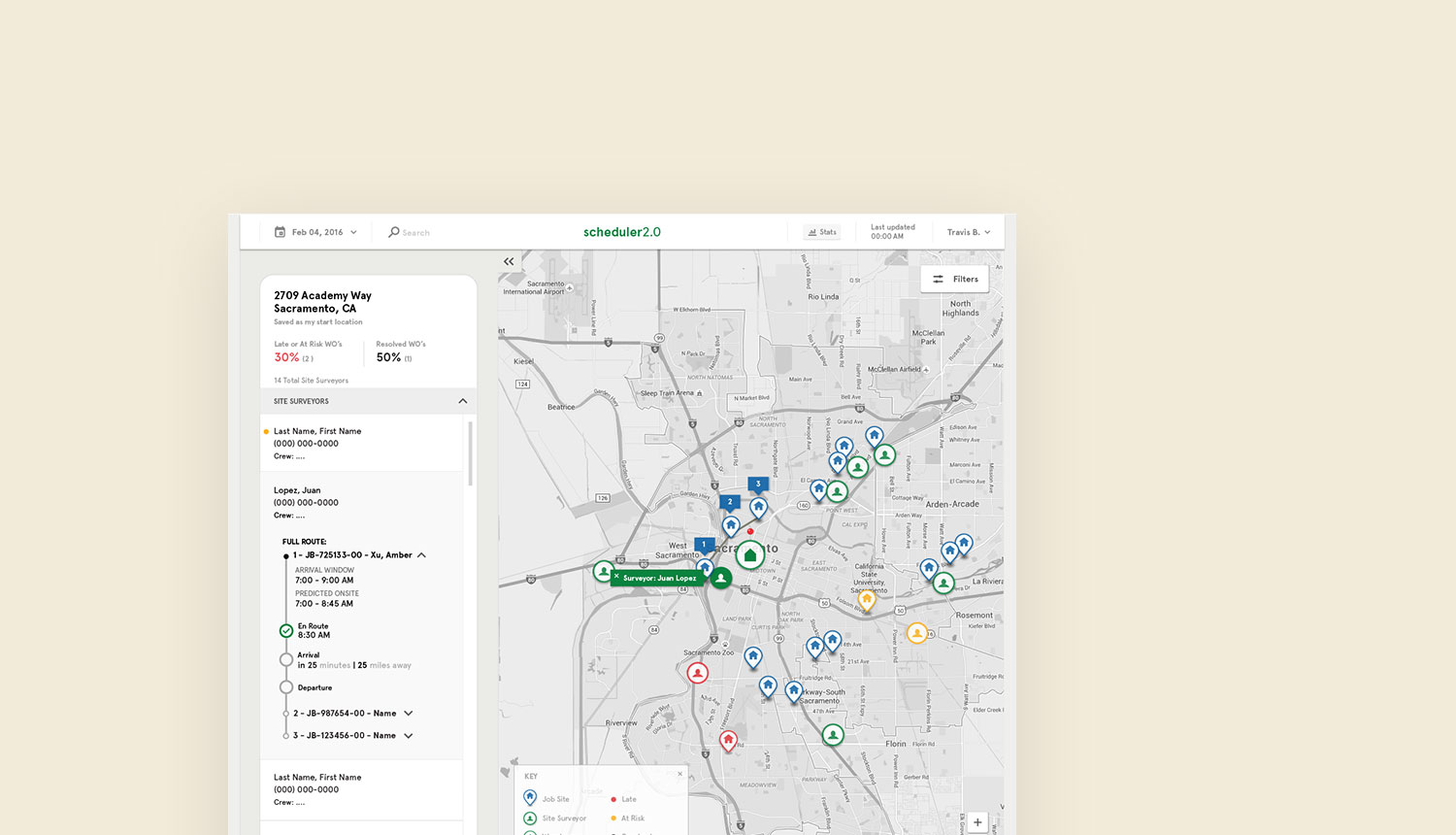This is a detailed image of a beige map background featuring various user interface elements and annotations. In the upper left-hand corner, there is a small calendar icon next to the date "February 4, 2016." To the right of this, there is a search bar adorned with a magnifying glass symbol, and further right, the text "Scheduler 2.0" appears in green lettering. The text "Stats" is located next, followed by "Last Updated" with a timestamp reading "00." Adjacent to this, the name "Travis B." is displayed.

In the lower left-hand corner, there is a white box containing the address "2709 Academy Way, Sacramento, California." Below the address, there are two percentages: "30%" in red and "50%" in another color. Underneath these percentages, the words "Site Surveyors" are present, accompanied by columns for "Last Name," "First Name," and a phone number, although the phone number is depicted as "0000000000." The box also mentions "Cover/Crew..."

Further down, another section marked "Full Route" shows detailed information: "XU Amber," an arrival window between 7 and 9 a.m., and an on-site prediction between 7 and 8:45 a.m. The status "Enroute" is marked next to a circle with a green checkmark, displaying "8:30 a.m." The subsequent labels "Arrival" and "Departure" follow, with "Arrival" shown next to a white circle. Below "Departure," some alphanumeric codes are listed, next to which the fields "Last Name," "First Name," and "0000000000" for the phone number are repeated.

On the map, there are color-coded circles and indicators. Blue dots mark job sites, green dots signify site surveyors, while red and yellow dots likely highlight other statuses or elements. One highlighted green icon, "Surveyor 1 Lopez," features a circle with a green house in the middle. Additionally, some blue houses (job sites) are numbered 1, 2, and 3.